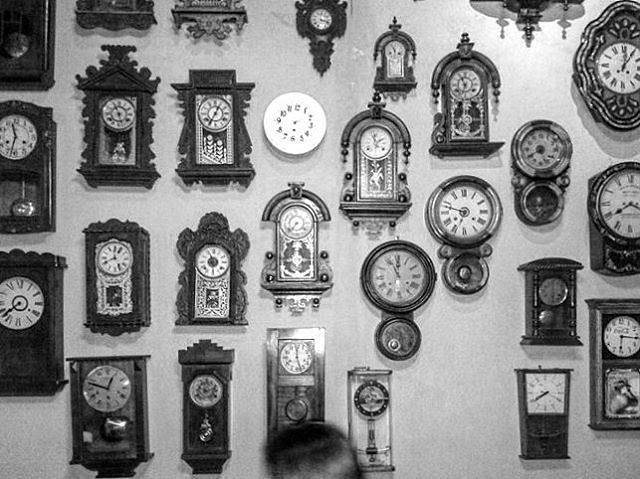This black and white photograph features a wall densely adorned with approximately 25 old-fashioned clocks of various shapes and sizes, giving the impression of a vintage collection. Most of these clocks are encased in ornate frames, resembling fancy picture frames, with some having squarish or rectangular contours while others boast rounded or arched tops, and a few embellished with a globe-like piece hanging below. Among this array of heavily ornamented timepieces stands one contemporary clock, a stark contrast with its plain white face and black numbers, devoid of any decorations. Some timepieces display Roman numerals, while others have standard numbers. The photograph is somewhat blurry, making it difficult to discern the exact time on most clocks. Hovering at the bottom center of the image is the slightly out-of-focus head of a man with patchy black hair, seemingly in motion and partially obscuring one of the clocks.